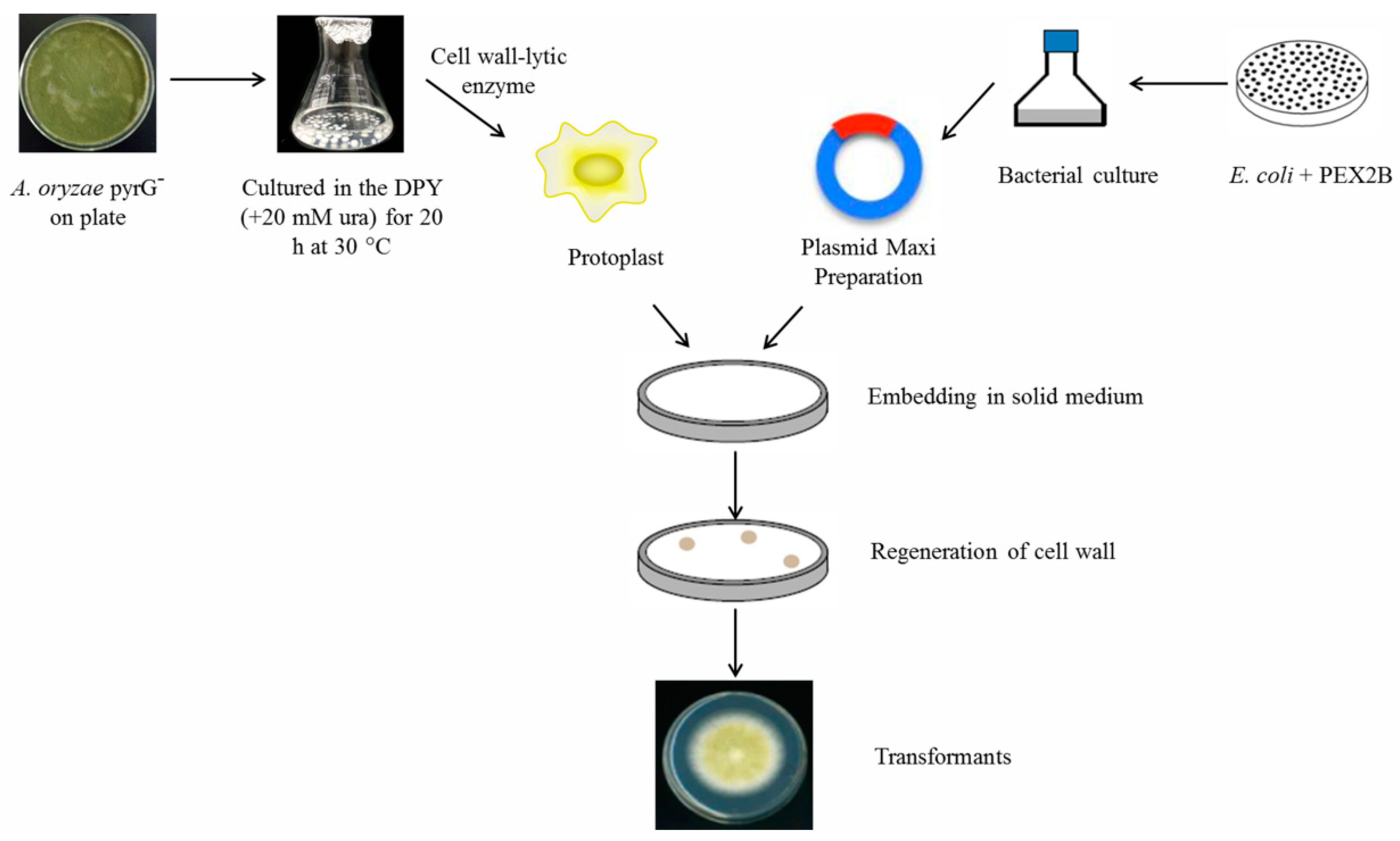This image is a detailed scientific diagram illustrating the transformation processes of bacteria, specifically E. coli combined with PEX2B. In the upper left corner, it shows a labeled petri dish indicating the presence of different bacteria or organisms, marked as "A, P, or G," and notes the culturing conditions: DBY plus 20 mm URA for 20 hours at 30°C. The diagram proceeds to describe several stages of bacterial manipulation, including:

- Cell wall lytic enzyme application to create protoplasts
- Plasmid maxi-preparation
- Embedding in a solid medium
- Regeneration of the cell wall
- Transformance

Several scientific objects, such as petri dishes and water beakers, are depicted throughout the diagram. A detailed observation reveals various textures and colors: a disk showing a white substance, another with clustered balls, and a third that's blue with yellow in the middle. The diagram advances through a Y-shaped pathway, illustrating how different components and stages integrate to transform bacteria effectively, with text primarily in Times New Roman font. The overall color scheme includes white, black, yellow, blue, and green elements, enhancing the visual clarity of each stage.